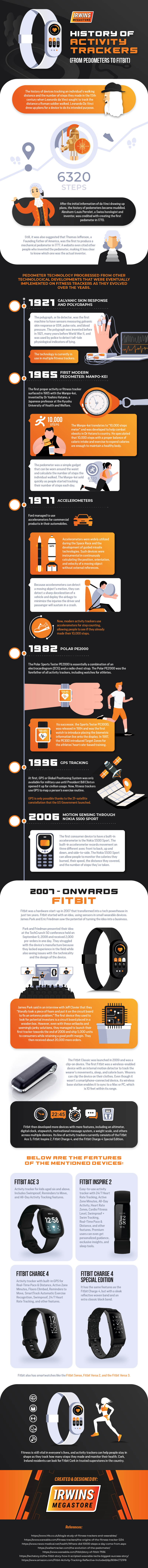The image is a narrow, film-strip-like banner ad for a Fitbit-style fitness tracker watch, primarily colored in orange, black, and white. At the top, there's a white watch displayed prominently, with bold orange lettering underneath. The ad features multiple screenshots illustrating various functions and activities the watch supports, such as physical activity tracking, charging methods, and environmental sensors. Additionally, it shows how the watch displays its charge status. Towards the bottom, there are three watches with black bands and the white watch featuring a cartoon-like figure jogging, emphasizing its fitness-tracking capabilities. The overall layout resembles a detailed step-by-step manual, with small, hard-to-read text providing instructions and highlighting essential features of the product.